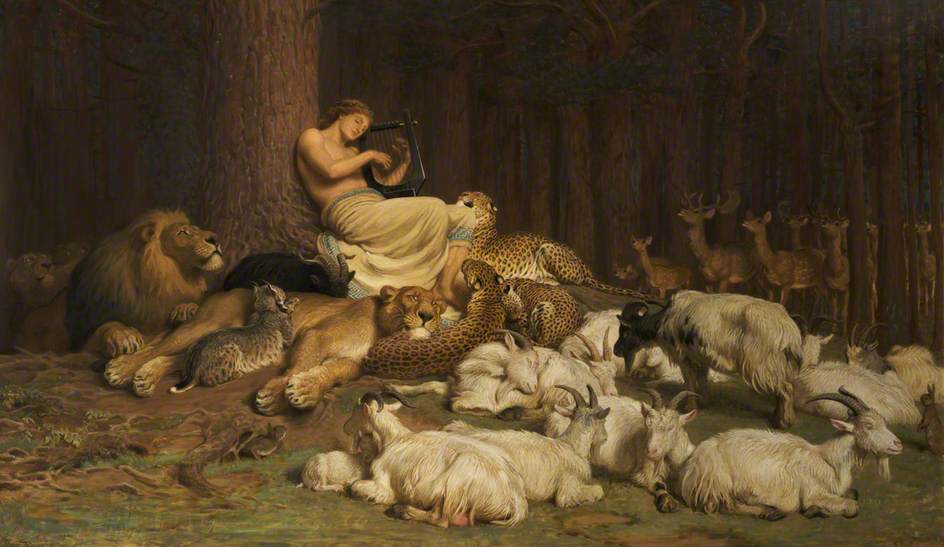This evocative oil painting, set outdoors at night, captures the mythological figure Apollo, identifiable by his brown hair and the small, black harp he holds delicately. Apollo, topless and clothed in a white robe bordered with blue, leans gracefully against a large brown tree trunk situated on the left-hand side of the composition. Surrounding him in a semi-circle are an array of animals, seemingly entranced by his music.

To Apollo's immediate right, a trio of leopards recline at his feet, providing a wild yet serene atmosphere. Behind the leopards, a lion and a lioness are captured in a tranquil moment; the lioness rests her head on one of the leopards' backs, while a bobcat nestles into the lioness. 

In the bottom right-hand corner of the image, several goats with curved horns lie on the grass, exhibiting a mix of restful poses—some gazing at Apollo, others looking away. Behind them, in the dense, dark woodland, a herd of about seven or eight deer stands transfixed by the music, heads alert and ears perked.

This detailed scene is further enhanced by patches of green grass in the foreground and an overarching darkness, imparting a sense of depth and nocturnal mystery to the setting. The absence of text allows the viewer to fully immerse in the tranquil, otherworldly interaction between the divine musician and his attentive animal audience.